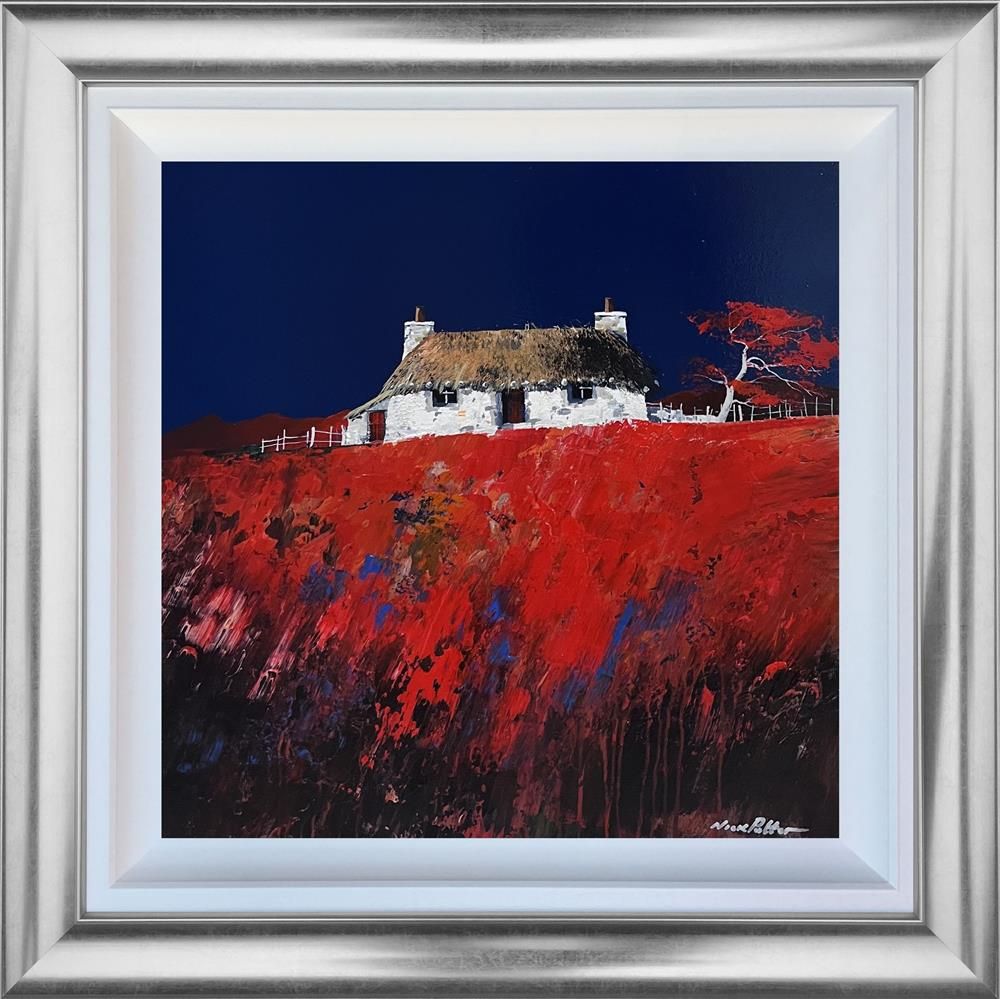This is a detailed painting encased in a grayish white, outer frame and white inner frame, portraying an old English-style country farmhouse. The farmhouse, characterized by its stone structure and distinctive thatched roof, stands prominently with its white walls and two prominent chimneys. The roof combines hues of brown and black, adding texture to the rustic dwelling. This painting captures the vibrant essence of its setting with primary, dark colors. The backdrop features a deep blue sky, contrasting but complementing the red earth and meadow depicted in the foreground. Surrounding the house is a white fence that encloses the property. On the right, a striking maple tree with vivid red leaves adds richness to the scene. The red flowers spread across the meadow leading up to the house enhance the pastoral beauty of the landscape. The painting is signed in white at the bottom right corner, though the signature is too small to decipher.